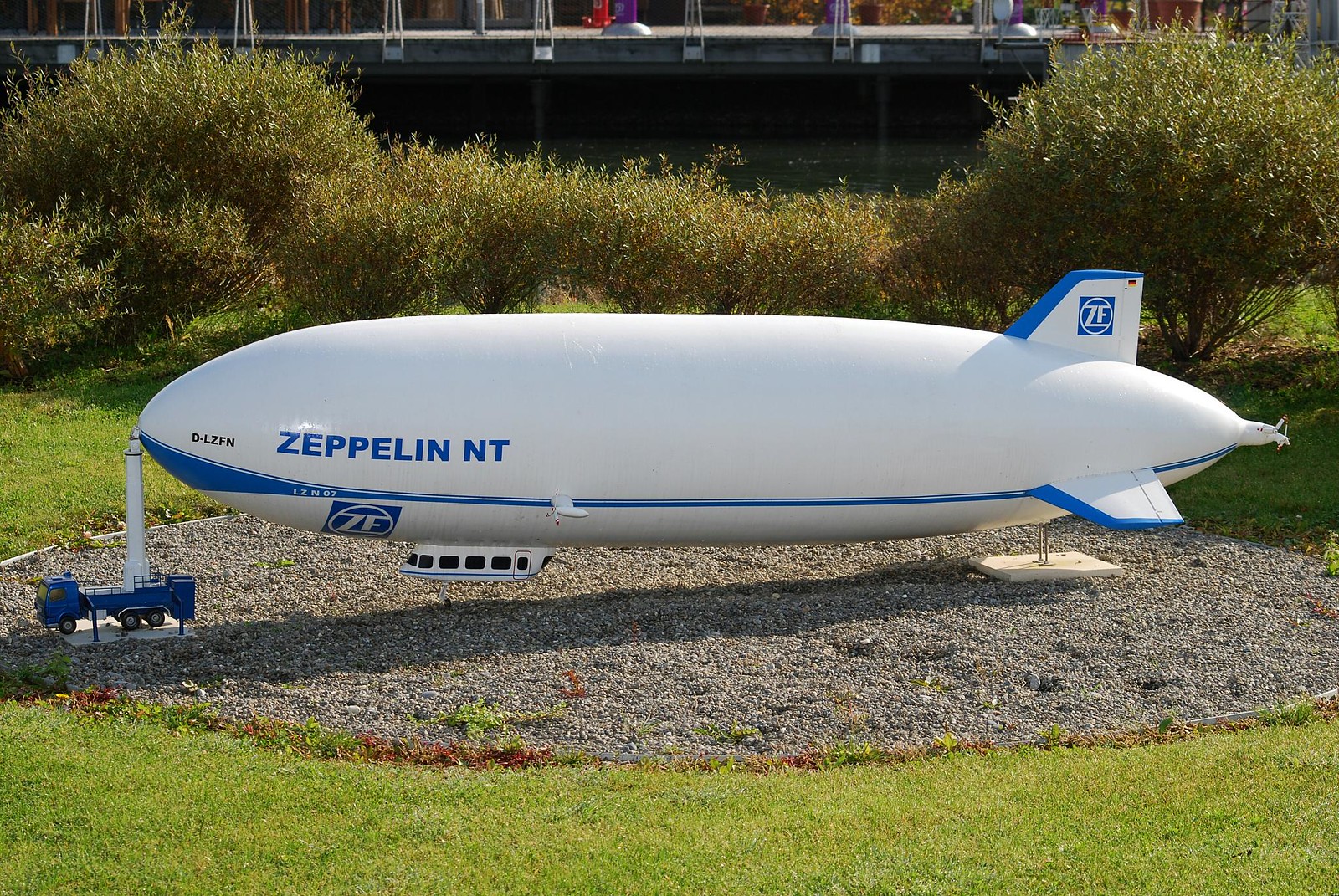In a picturesque outdoor scene on a sunny day, this landscape-oriented photograph showcases a miniature white Zeppelin with blue accents, prominently displayed on an oval dirt patch encircled by lush green grass. The Zeppelin, marked with "Zeppelin NT" in bold blue letters and adorned with blue-edged fins bearing a "ZF" logo, is positioned to the left, its tail extending to the right. A toy blue truck with a supporting pole at its front is attached to the Zeppelin’s nose, resembling it towing the airship. The scene is enhanced by manicured shrubs in the midground and the partial view of a serene river and a small bridge in the backdrop, suggesting a tranquil park-like setting.